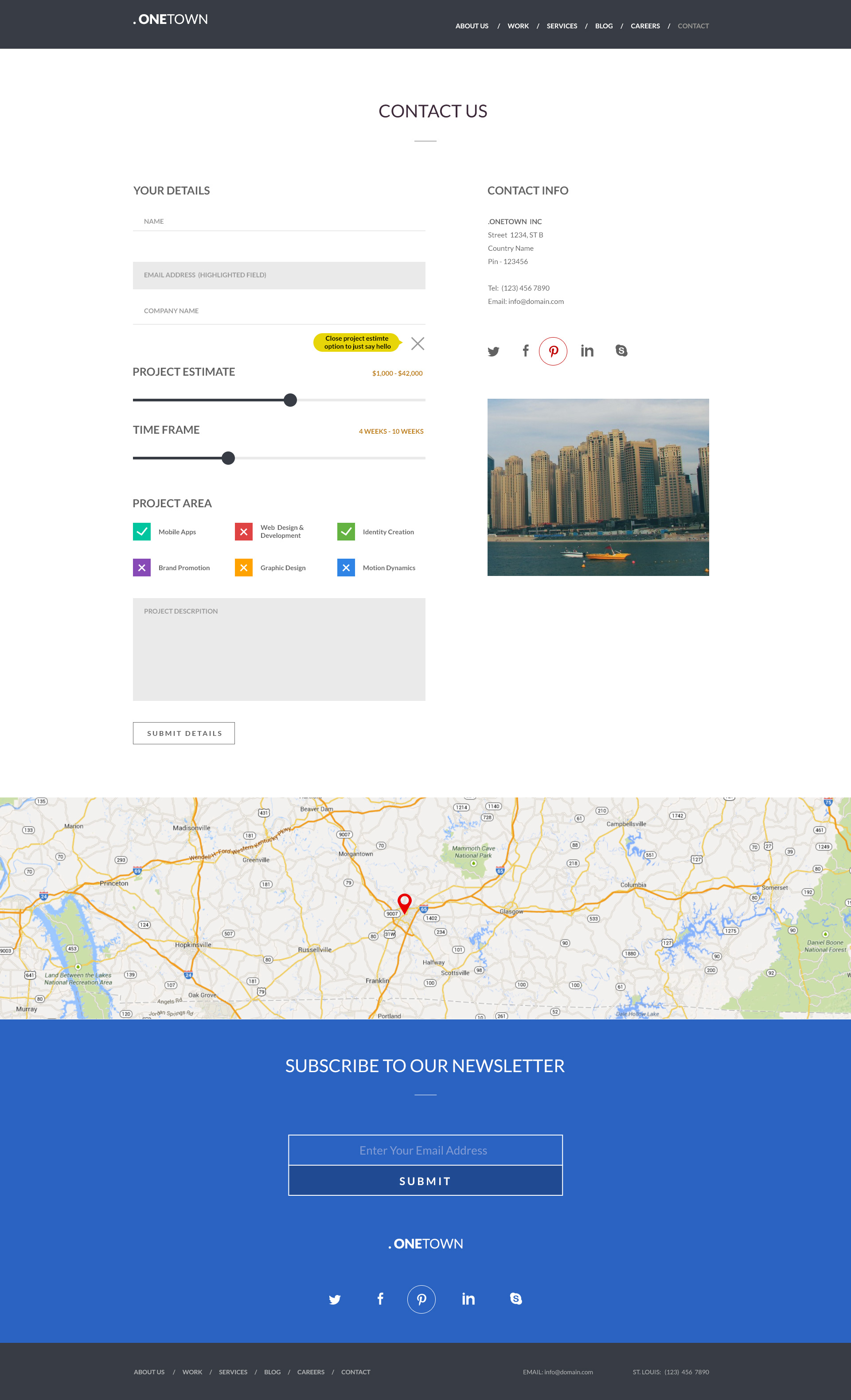This digital image, sourced from the OneTown website, captures a stunning view of a large city situated along a waterfront. An orange boat is prominently featured on the water, adding a vibrant touch to the serene landscape. The composition is enhanced by the presence of various navigational elements and contact information, including a "Contact Info" button that directs users to OneTown, Incorporated. Their address is listed as 1234 Street B, with the country and postal code specified as well as their telephone number (123-456-7890) and email (info@domain.com).

Social media icons for Pinterest, Facebook, and Twitter, the latter depicted with a little bird icon, are also visible, suggesting avenues for engagement. An accompanying map highlights several notable locations, such as Mammoth Cave National Park and towns including Morgantown, Scottsville, Franklin, Portland, Columbia, Campbellsville, Greenville, Russellville, Madisonville, Hopkinsville, Oak Grove, Princeton, and Marion. The image also incorporates an option to subscribe to the newsletter, inviting viewers to stay updated with the latest information and developments.